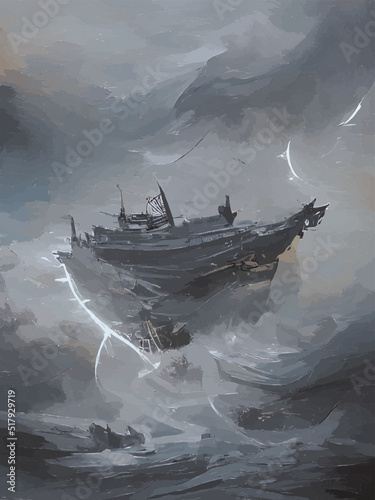The image is a rectangular drawing measuring approximately three to four inches tall and two to three inches wide, depicting a large ship navigating through a violent ocean storm. The ship itself appears to be a blend of a pirate ship and a cruise ship, moving from the left-hand side towards the right. It is portrayed in dark grays with intricate details that hint at an older design, possibly with sails.

The turbulent waves are colored in a spectrum of dark and light grays, with some hints of red, violet, and purple, adding a dramatic, violent effect. These colors are mirrored in the stormy sky, suggesting the presence of lightning amidst the chaos. There are occasional touches of brown and blue in the sky, contributing to a blocky and textured appearance.

In the bottom left corner of the illustration, there is a watermark in white print, reading "Adobe Stock A517-929-719." Additionally, a transparent watermark with the text "Adobe Stock" is diagonally sprawled across the entire image, providing a subtle overlay that runs from the lower left to the upper right.